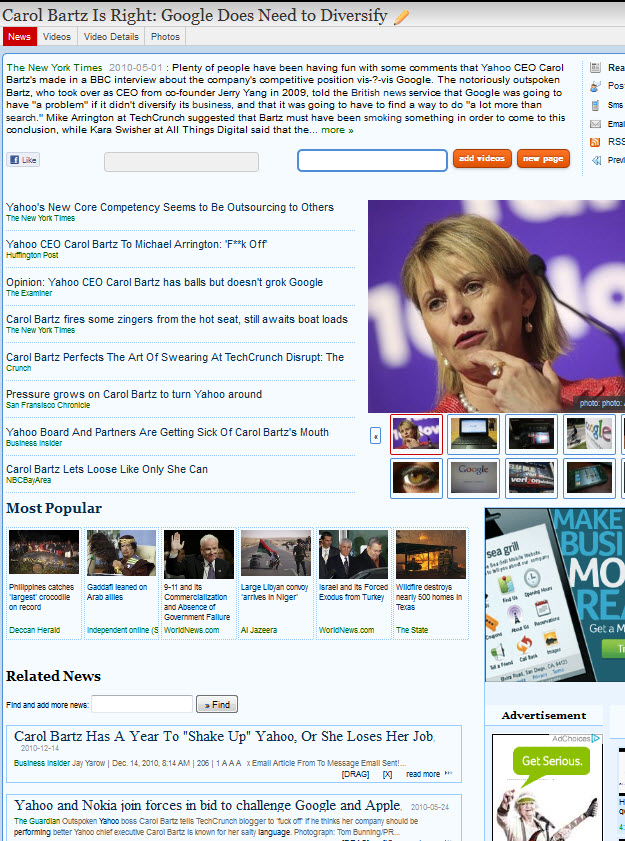The image is a desktop screenshot of a website focused on a news article titled "Carol Bartz is right. Google does need to diversify." The browser's address bar and type are not visible. The website features several navigational tabs including News, Videos, Video Details, and Photos. The central content of the page showcases an article from The New York Times dated May 1, 2010. The article discusses comments made by Yahoo CEO Carol Bartz during a BBC interview, emphasizing Google's need to diversify beyond its search business.

Carol Bartz, known for her outspoken nature since taking over as CEO from Yahoo co-founder Jerry Yang in 2009, warned that Google would face significant challenges if it didn't expand beyond search. The article mentions various reactions to Bartz's interview, including critical remarks from Mike Arrington of TechCrunch, who sarcastically suggested that Bartz must have been under the influence to arrive at such a conclusion, and Kara Swisher from AllThingsDigital, whose full comment is partially obscured by an ellipsis.

The webpage also displays a Facebook-like icon and features areas for adding videos or new pages, indicated by two blank bars. Below the main article, the page lists popular headlines, presumably related to the central theme of Yahoo, Google, and YouTube, along with advertisements. Further down, related news continues the focus on Carol Bartz and her comments. The dated design of the website reflects web aesthetics from 2010, highlighting how much web design has evolved since then.